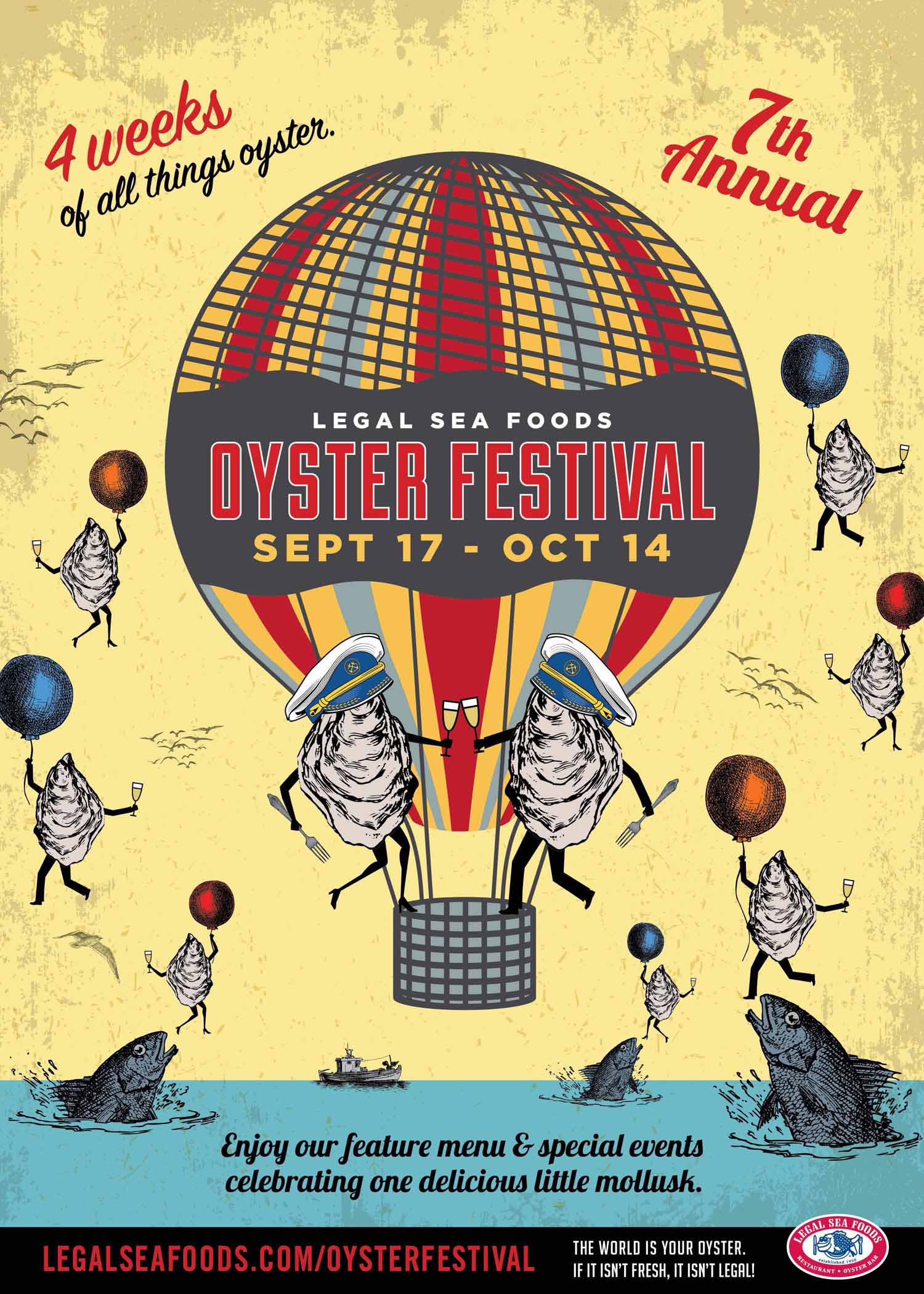This poster advertises the seventh annual Legal Seafoods Oyster Festival, running from September 17th to October 14th. Dominating the center is a large hot air balloon striped in red, yellow, and blue. The balloon displays the festival's title, accompanied by phrases like "Four weeks of all things oyster" and "The world is your oyster. If it isn't fresh, it isn't legal."

In the balloon's basket, two oysters, anthropomorphized with legs, arms, captain's hats, and forks, joyously clutch champagne glasses. Surrounding this whimsical scene are smaller oysters, each holding a balloon and a glass of champagne, soaring above a stylized blue ocean teeming with fish. In the background, a classic fishing boat adds to the maritime theme. The entire design is rendered in a charming vintage style, creating a festive invitation to the event. The poster concludes with a call to visit LegalSeafoods.com/OysterFestival for more details.